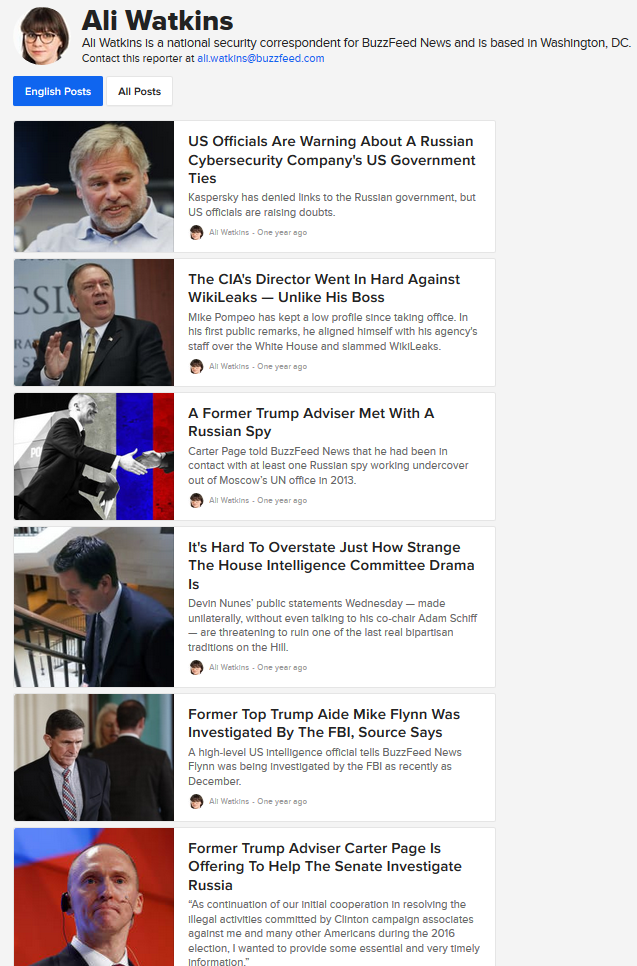At the top left of the image, a circular user icon features a woman with brown hair and bangs. She is wearing thick black-rimmed glasses with large round lenses, and she has red lips and an olive skin tone. To the right of the icon, in bold black lettering, the name "Allie Watkins" is displayed. Below this, in smaller, non-bold, black sans serif font, it reads: "Allie Watkins is a national security correspondent for BuzzFeed News and is based in Washington, DC." The reporter's contact, in blue text, is "allie.watkins@buzzfeed.com."

There are two tabs beneath this section. The first tab on the left is a blue rectangle with white text that says "English Post," indicating it is selected. To the right, a white rectangle contains the text "All Posts" in black.

The image also displays a thumbnail of a man with gray hair, holding up his right hand with all fingers extended except his thumb. He is wearing a light blue button-up shirt and has a gray mustache and beard. To the right of this thumbnail, in black text, is the headline: "US officials are warning about a Russian cybersecurity company's US government ties."

Below this, another thumbnail shows a man standing in front of a sign. He has his left hand raised with all fingers spread and his palm facing the audience. He is dressed in a black suit with a white undershirt and a yellow tie featuring a black design. The background has a gray sign, and the man appears surprised. The headline for this segment, in black text, reads: "The CIA's director went in hard against WikiLeaks – unlike his boss."